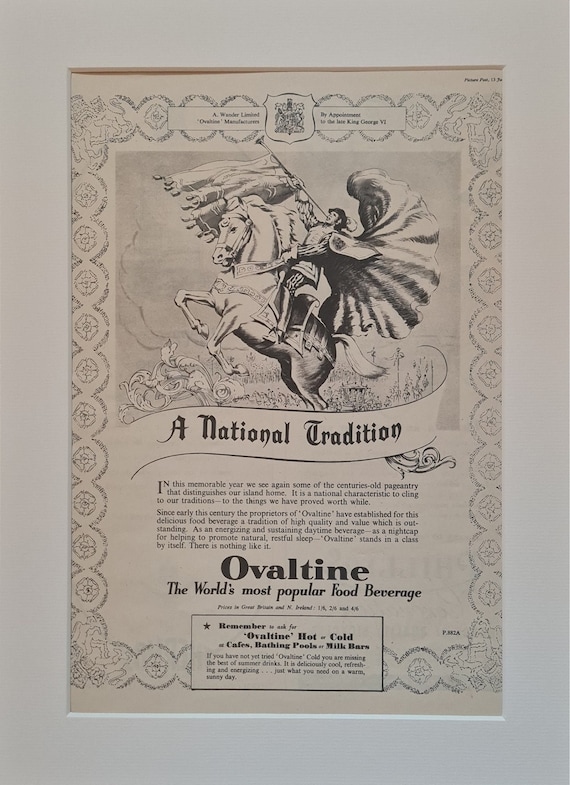This image is an antique advertisement for Ovaltine, prominently showcasing a dramatic illustration of a man clad in armor and boots, riding a horse that is rearing on its hind legs. The man is blowing a long trumpet adorned with a streaming banner, his cape dramatically billowing in the air, and his hat decorated with a feather. The bold text at the top of the flyer reads, "A National Tradition," highlighting the enduring cultural practices that define the island home featured in this ad. The central text elaborates on the centuries-old pageantry and underscores Ovaltine's high quality and value, establishing it as an energizing, sustaining daytime beverage and a nightcap promoting restful sleep. The advertisement asserts the unique position of Ovaltine, stating, "Ovaltine stands in a class by itself. There is nothing like it." Further emphasizing its popularity, the ad boldly declares, "Ovaltine, the world's most popular food beverage." Towards the bottom, it encourages consumers to "ask for Ovaltine, hot or cold, at cafes, bathing pools, or milk bars." Additional, unidentified text is also mentioned beneath the main body of the advertisement.